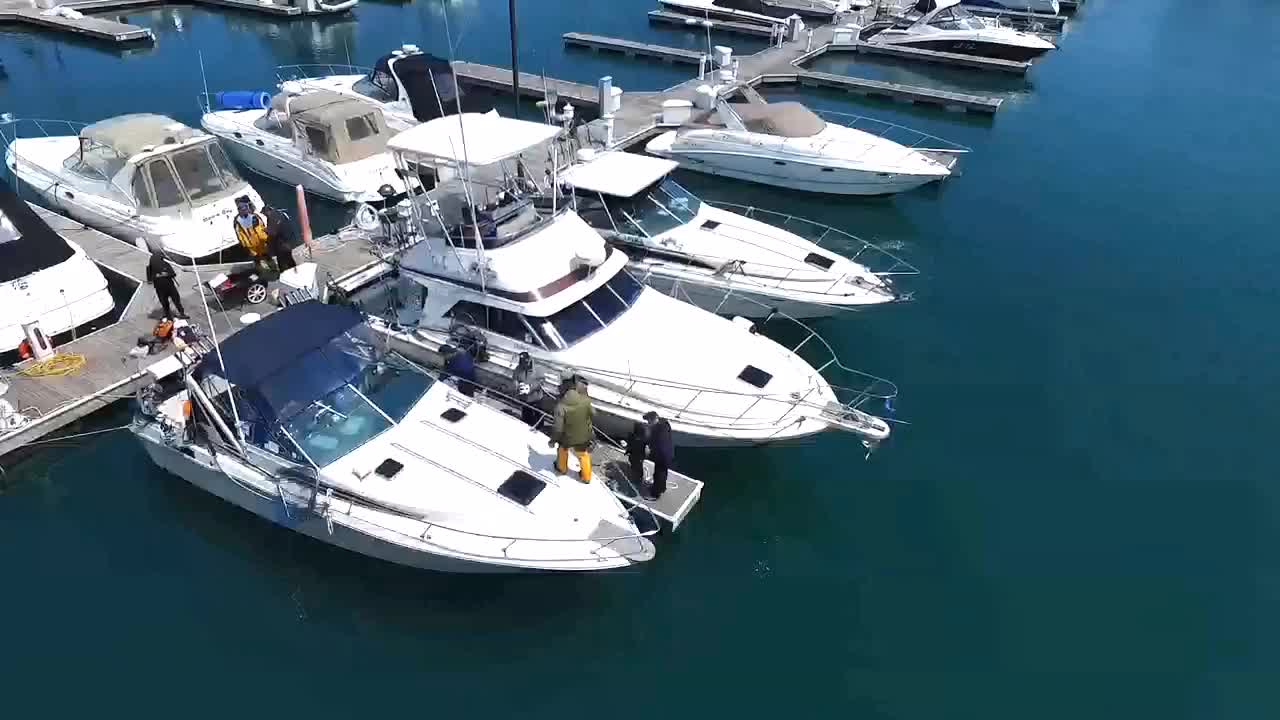This detailed color photograph, taken from a slightly elevated angle, captures a vibrant scene at a marina dock where numerous boats are moored. The setting is defined by exceptionally calm, blue-turquoise water that lends an almost surreal, smooth backdrop to the image. Five yachts and power boats line the right side of the central wooden pier, which is characterized by gray horizontal slats. These larger vessels extend from the top right through the center, down to the very left, holding prominence in the composition. On the left side, there are three smaller vessels, potentially white boats with gray tarps, clustered nearer to the top left corner.

Four figures animate the scene: one stands out in a gray-green coat and yellow pants on the bottom-right yacht, seen only from behind. The other three are dispersed along the dock; two in dark coats, and one in a distinguishable yellow sailing jacket, a key visual cue. Beside this person is a yellow rope and a wagon, adding functional elements to the atmospheric setup. This photograph intricately links the tranquility of still waters and the activity of a bustling marina, portraying both the serene and the industrious facets of dock life.